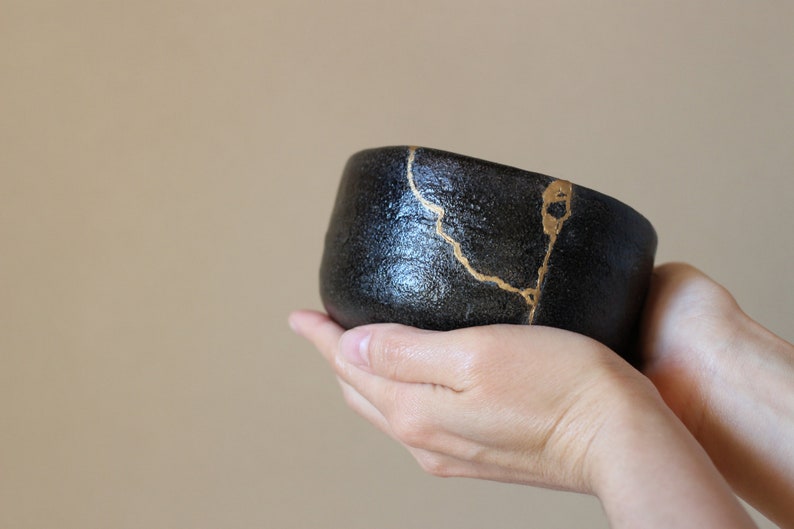In a horizontally aligned, rectangular photograph with a solid beige background tinged with brownish-gray, a woman's cupped hands extend from the bottom right corner towards the center, holding a large, round, black, and shiny object. The object, which fills her palms and partially obscures the view of her wrists and fingers, appears to be made of stone or metal, exhibiting a textured, pebbled surface. Prominent golden markings detail the object—a vertical line from top to bottom, and a second, curved line descending diagonally from the top left. Additionally, there is a light brownish splotch and some swirls that create an intricate design above the base of the woman's thumb. The light, seemingly natural, illuminates the scene from the left, casting a bright and cheery glow over the entire image.